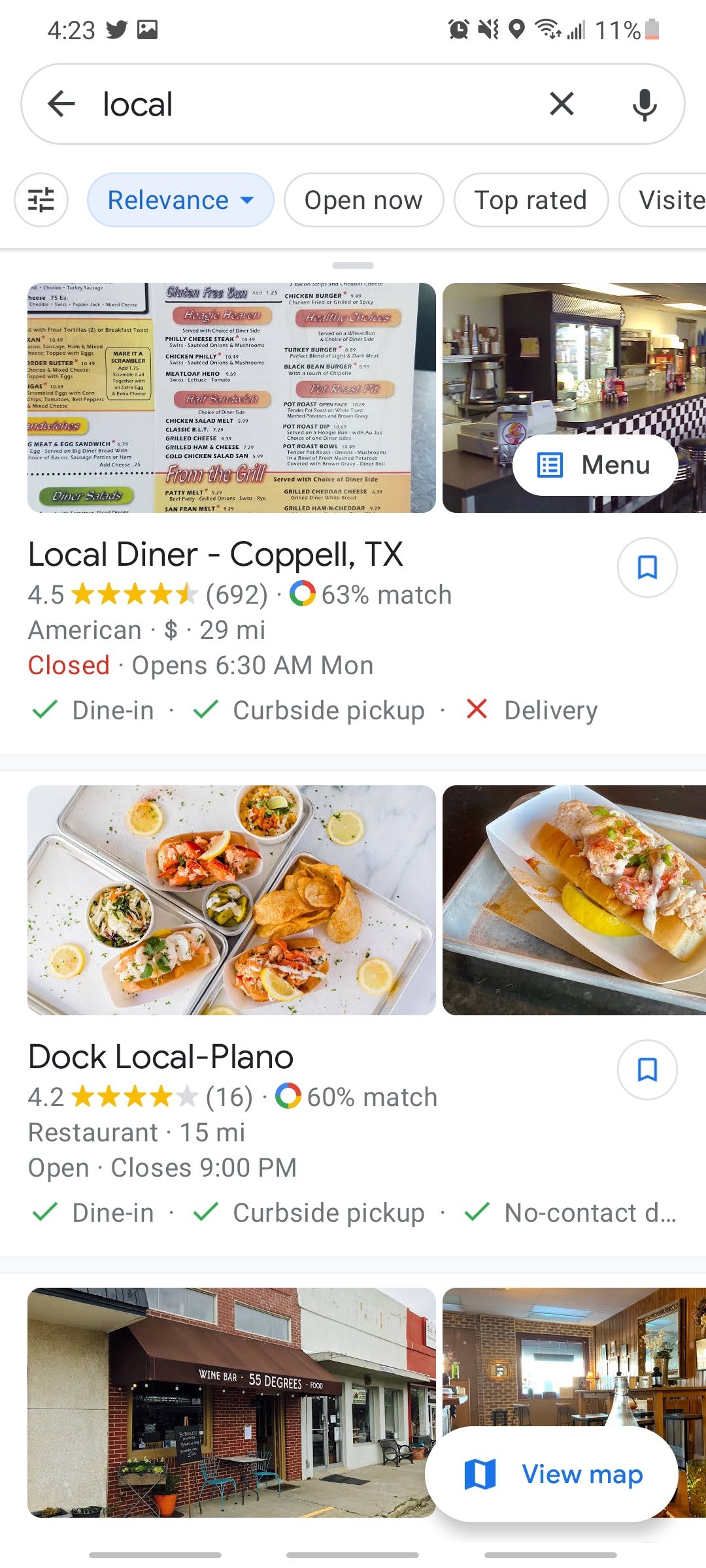In this screenshot set against a solid white background, we are viewing what seems to be a snapshot from a cell phone screen. The top left corner features dark blue text displaying the time as "4:23," alongside a series of icons: a Twitter icon and a photo gallery icon. On the upper right corner, several icons appear, including an alarm clock, a notifications-off symbol, a map icon, Wi-Fi status (showing it is on), and a battery icon indicating an 11% charge remaining.

Beneath these elements, a search bar is visible, displaying the word "local" with an arrow pointing to the left. Nested below the search bar are the search results. The first result is for a "Local Diner" located in Coppell, Texas. This entry includes two photos: one in color depicting the diner's menu, and another showing the interior of the diner. The establishment boasts a rating of 4.5 stars, with the stars presented in yellow and a total of 692 reviews. It is classified as American cuisine, marked with a single dollar sign indicating cheap pricing, and it is located 29 miles away. The status of the diner is marked as "closed" in red text.

Below this listing, another restaurant, "Doc Local" in Plano, is featured. It has a 4.2-star rating, but details such as the number of reviews, type of cuisine, price range, and distance are not provided in this partial view.